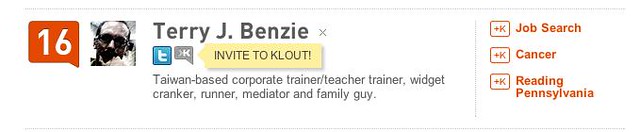The image appears to be a snapshot of a website, possibly from a friendship or dating app, featuring a profile. Dominated by a white background, the layout includes a variety of colored elements. In the top left corner, there's a small red square with the number "16" in white print beside a photograph of a man. To the right of the photo, the name "Terry J. Benzie" is prominently displayed. Directly below his name, on a yellow background, are the words "Invite to Clout." Toward the right side of the image, text in red print lists "Job Search," "Cancer," and "Reading, Pennsylvania." Additionally, Terry's detailed profile highlights him as a "Taiwan-based corporate trainer, teacher, trainer, widget cranker, runner, meditator, and family guy." The overall style is indicative of a modern website interface with a horizontal rectangular design structure.